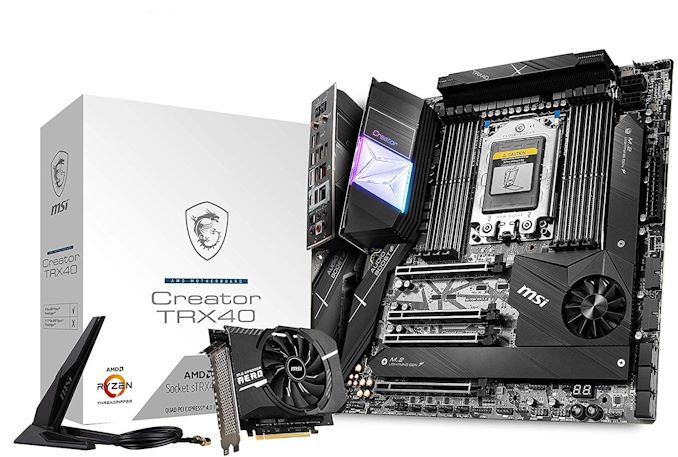The image showcases a detailed view of a high-end computer graphics card and its packaging. On the left side of the image, there is a box from AMD Ryzen, prominently labeled "Creator TRX40," which indicates it houses components for powerful computational tasks. The box is primarily white and features the MSI logo, characterized by a shield with a dragon inside. Adjacent to this, on the right side of the image, the main focus, the graphics card, is displayed. This card, made by MSI, is a sophisticated device with intricate components and is labeled "Aero." It is designed to be inserted into a computer and features a black and silver color scheme. The graphics card appears to have various components, including a cooling fan to prevent overheating and numerous ports and connectors for optimal performance. A monopod in black and silver is also present on the right, labeled with the red letters "MSI," and a hand is visible near this writing. The overall appearance of the setup is sleek, with various shades of gray and black, indicating this is a robust and efficient model suitable for handling demanding programs and tasks.